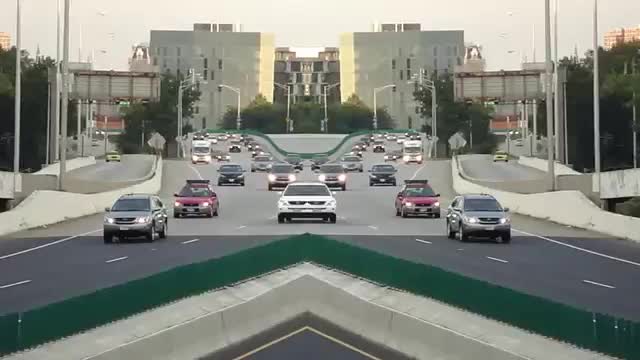The image depicts a symmetrical, mirrored highway scene where cars are driving towards the viewer. The road is at the center, divided by a green triangular median with a grey triangle inside it, creating a symmetrical split that extends to the bottom left and right corners. The central focus is a white SUV mirrored at the center, with a grey SUV in front of it and a red car behind it, along with a taxi in an adjacent lane. More indistinct vehicles follow behind. In the background, uniform white buildings with black elements on their rooftops are visible, accompanied by trees and various streetlights. The image emphasizes symmetry, with the left half mirroring the right, creating a highly structured and repetitive visual effect.